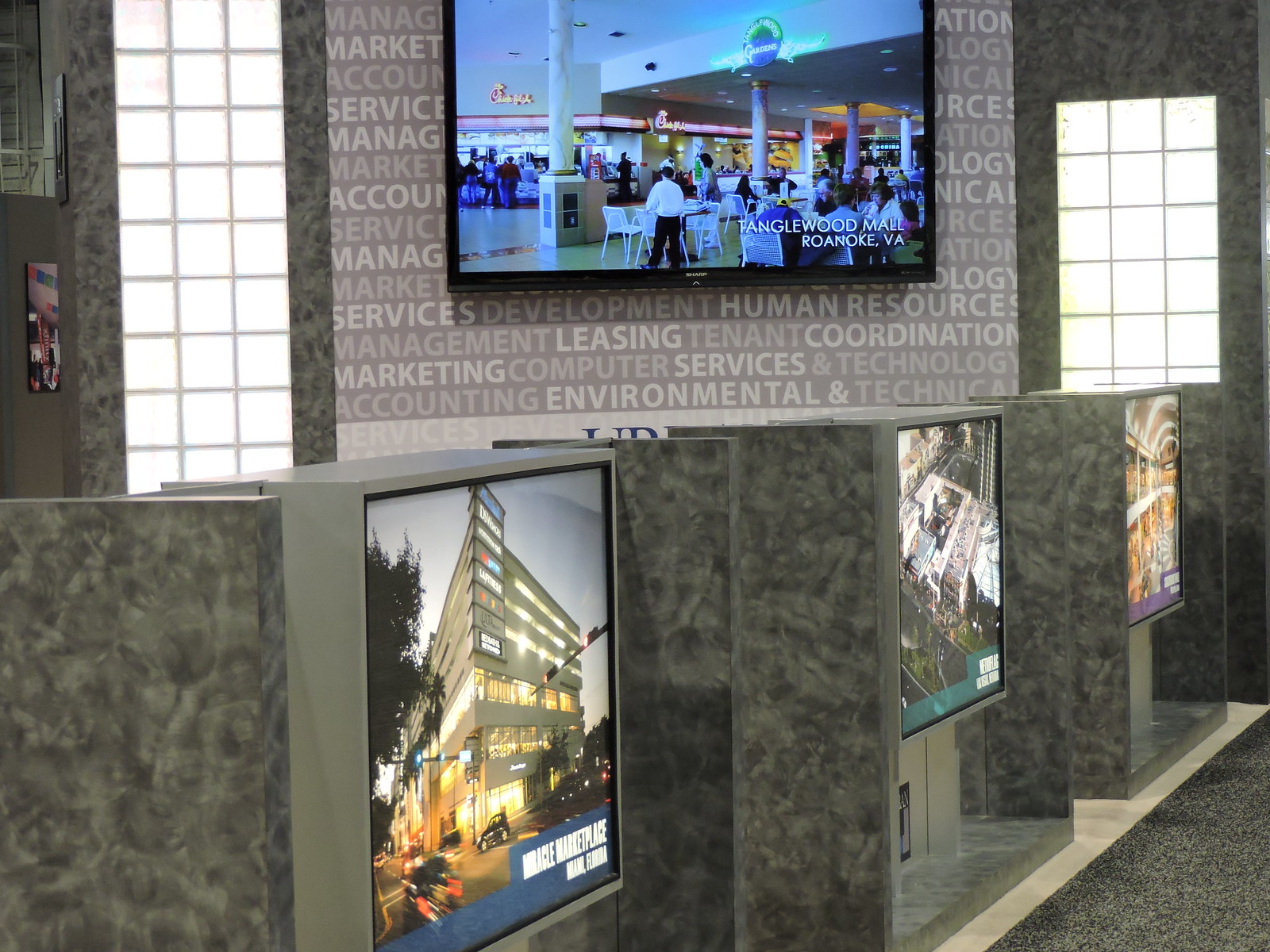The image depicts a sophisticated lobby or waiting area, likely belonging to a real estate company or business office, characterized by a predominantly gray color scheme. The background wall features multiple words like "management," "leasing," "tenant," "coordination," "marketing," "computer services and technology," "accounting," and "environmental and technology," inscribed in faint light-colored text. Mounted on this gray wall is a TV displaying an image of a bustling food court inside a mall, notably featuring a Chick-fil-A among other eateries, with numerous people seated and dining.

Flanking the TV are two tall windows with a grid of small square panes; the left window extends from the top of the image downward, partially obscured by items in the foreground, while the right window has some wall space above it. Below, the foreground reveals a row of three cabinets arranged from the bottom left diagonally upwards to the right, each featuring glass fronts and marble-like sides though not actual marble. These cabinets house monitors on their tops, with the clear image of a building on the leftmost monitor that includes white text on a blue strip beneath it, whereas the other two monitors display indistinct images. The cabinets appear to sit on a slightly raised light-colored platform above the speckled gray and black carpet, suggesting a polished and modern aesthetic for the space.